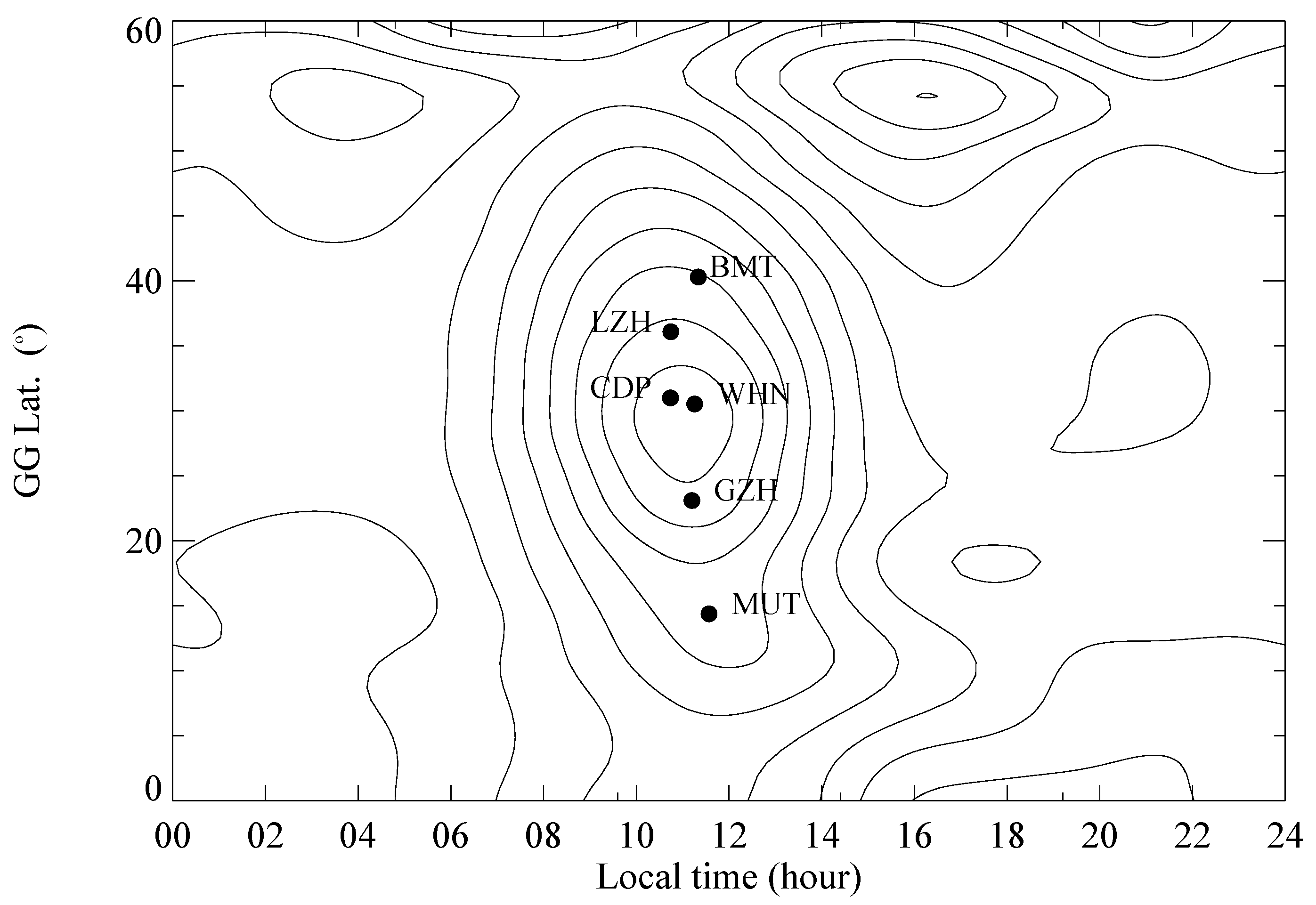This image is a black-and-white scatter plot, presenting a detailed diagram with concentric circles creating ripple-like patterns akin to those seen on a lake. The x-axis is labeled "local time and hour," ranging from 0 to 24, while the y-axis is marked "GGLAT," likely representing degrees of latitude, extending from 0 to 6. Positioned within this graphical spread are several black dots, each denoted by abbreviations such as BMT, LZH, CDP, GZH, and MUT, suggesting specific locations. These dots, placed mainly in the center of the plot, might indicate events or data points relevant to different latitudes and times, possibly hinting at phenomena like earthquakes occurring at particular times and latitudes. The image functions as an informational graph showcasing the intricate relationship between local time and latitude.